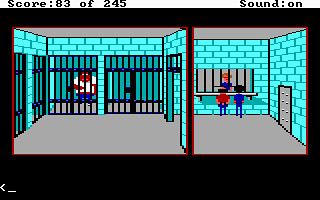In this vibrant 8-bit style game scene, an aqua blue brick jail is depicted with intricate details. The jail features four cells, one of which houses a large man wearing a white shirt and blue pants. The jail is divided by a center wall with an archway. To the right of the archway, a police officer is inset within the wall. Nearby, there is an office space where another cop with bright orange hair is situated. This cop is engaged in conversation with two individuals, one to his left sporting a red shirt and black hair with a bald spot, and another to his right wearing a blue shirt and black hair.

The jail cells are secured with black bars, and a notable gray steel door with visible rivets is set into the aqua-colored brick wall, adding to the robust, industrial atmosphere. Along the top of the screen, a white bar indicates the game's current score, showing "Score: 83/245" in black text. It also displays the sound status as "Sound: On." At the very bottom left corner, there is an "X" followed by a small dash, suggesting a possible text input or command prompt area.